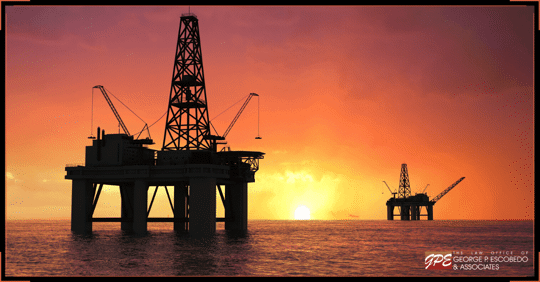The image captures two oil rigs silhouetted against a mesmerizing sunset over the ocean. The sky is awash with a warm palette ranging from deep purple and red in the upper corners to a brilliant yellow near the Sun, which is setting on the horizon. The oil rigs, constructed with tall, triangular metal structures resembling an Eiffel Tower-like lattice, stand on massive concrete pillars. Each rig is equipped with two large cranes positioned on their sides. The prominent rig is situated in the left center of the image, towering up to the top, while a smaller, more distant oil rig occupies the middle background. The ocean spans the lower portion of the photo, reflecting the sky's vibrant colors. Completing the composition is a black border around the image, with the name "George P. Escobedo and Associates" in white at the bottom right.